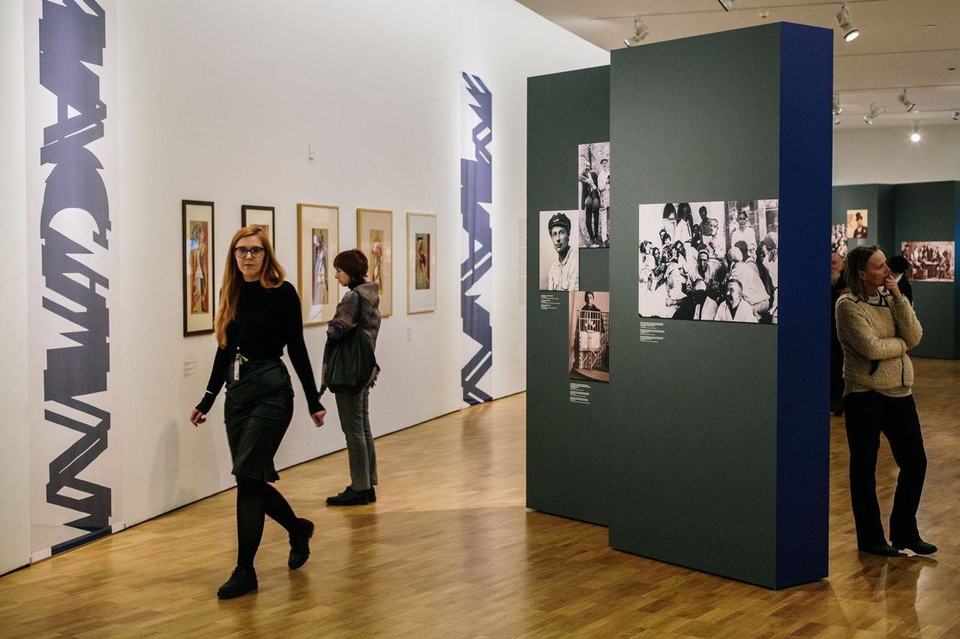This photograph captures a vibrant scene within a well-lit art gallery exhibit. In the foreground, two standalone walls are adorned with black and white and sepia-toned photographs, possibly depicting navy men and other individuals, including one wearing a top hat. The left wall in the background showcases an array of paintings, contributing to the gallery’s diverse collection of media. Several visitors are present in the scene: a woman, possibly the curator, equipped with a microphone is looking towards the camera, while another woman behind her and a third to the right both appear to be thoughtfully engaging with the artwork. The gallery features a traditional wooden floor, typical of such settings, enhancing the formal yet inviting atmosphere. The mix of paintings and photographs along with the thoughtfully placed moveable walls allow patrons to immerse themselves in a rich and varied artistic experience.